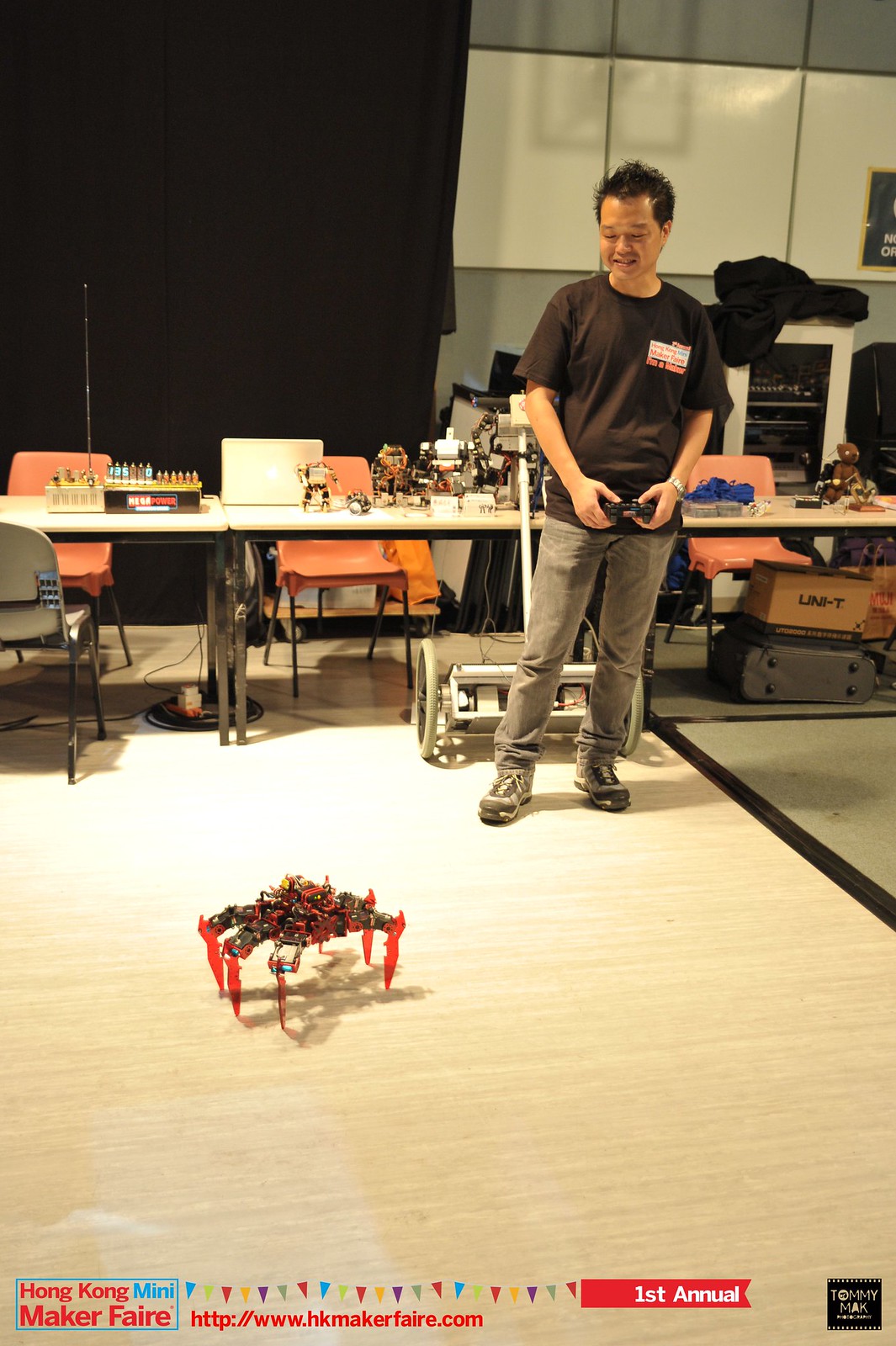In this color photograph, a man, who appears to be about 45 years old with short spiky black hair and dark skin, stands in the top right corner of the image. He is smiling and looking down as he uses a remote controller to operate a small, intricate robotic creature. The spider-like robot, positioned on the bottom left of the wooden floor, boasts six pointed red-orange legs and a complex black top, reminiscent of a mother spider carrying baby spiders. The man, dressed in a brown shirt with the "Hong Kong Mini Maker Faire" logo and wearing beige khaki pants and sneakers, stands in an environment set up for a technological event.

Behind him, the room features gray walls with some white panels, a long row of white desks laden with various mechanical robots and remote-controlled devices, and orange chairs arranged behind the tables. A black curtain is visible on the left side of the image. Adding to the informative nature of the photo, a blue rectangle with red text at the bottom reads "Hong Kong Mini Maker Faire," accompanied by the event's website URL, and a banner announcing it as the "First Annual" fair. This promotional shot effectively captures the blend of innovation and enthusiasm characteristic of the Maker Faire environment.